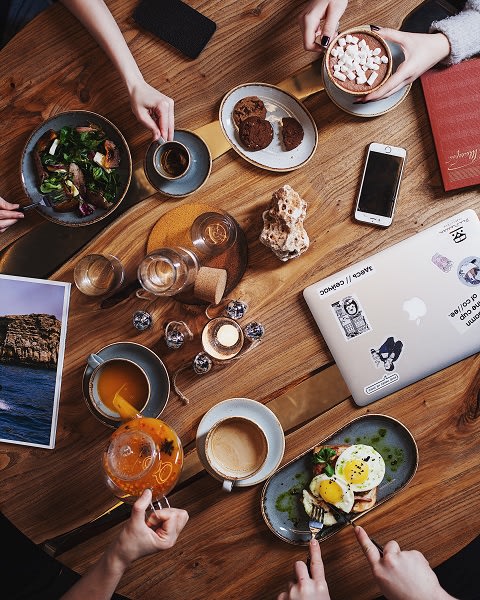This image, a color photograph oriented in portrait, showcases an overhead view of a bustling wooden table, notably oval in shape. Various hands converge from different directions, indicative of at least four people engaged in a casual dining or meeting scenario. The hands at the bottom right are cutting into a fried egg resting on an oval blue platter, while nearby, a clear glass teapot pours amber-colored tea into a white teacup from the left. To their left, a pair of hands is also occupied with a teacup and saucer. 

On the top left, hands are seen eating from a blue bowl of salad and lifting a cup of tea from a matching blue saucer. Adjacent to this, at the top right, hands cradle a large mug topped with marshmallows, likely a hot chocolate, and a plate of brown cookies sits in front of them. The table also holds a silver laptop adorned with stickers, a phone, a book, and various other small items such as candles and a rock, adding to the sense of a busy scene with much going on. Light filters into the indoor setting, enhancing the warm and convivial atmosphere captured in this photograph.